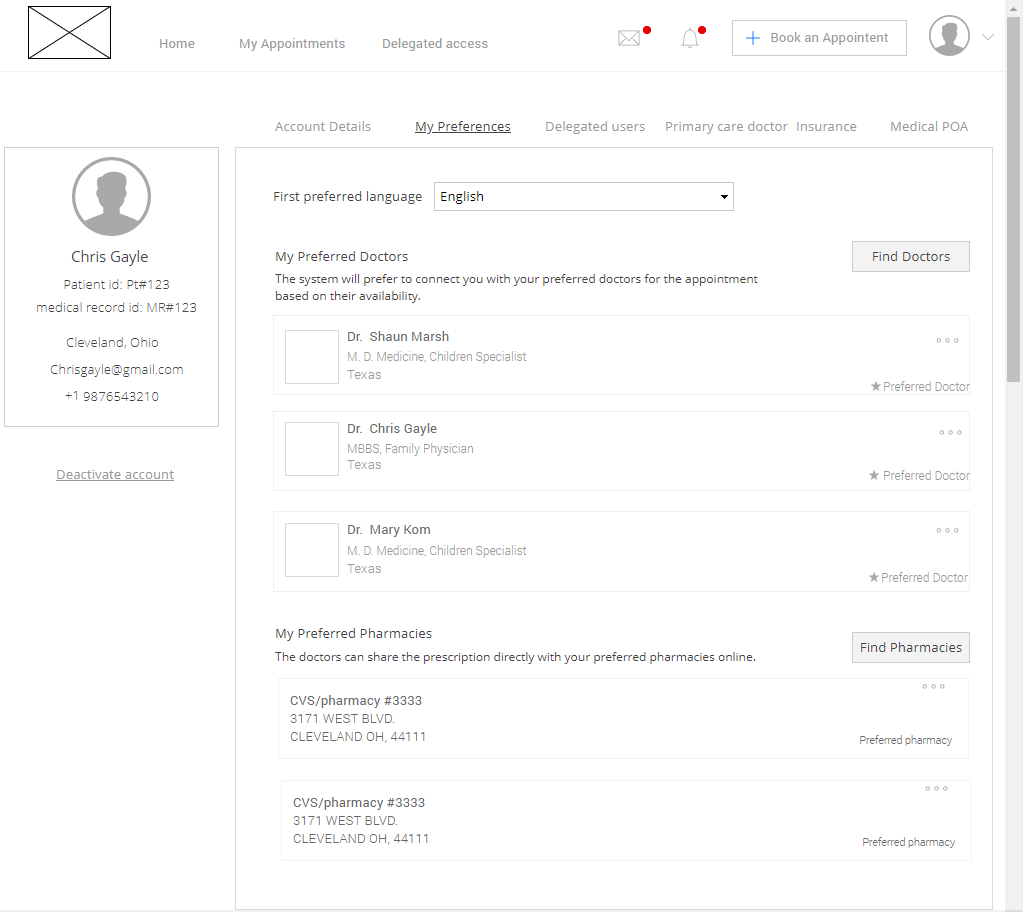This image showcases a detailed page from a patient's medical records interface. At the top left, there is an icon of an envelope. Directly below this, in a left-aligned column, is a circle featuring a person icon. Underneath this icon, various details about the patient are listed: the name "Chris Gale," a patient ID number, a medical record ID number, the location "Cleveland, Ohio," the patient's email address, and phone number. Below these details, there is an option labeled "Deactivate Account."

A banner stretches across the top of the page featuring navigation options: "Home," "My Appointments," and "Delegated Access." Accompanying this banner are icons of an envelope and a bell, both marked with red dots, and a tab labeled "Book an Appointment."

Just beneath this banner, a secondary menu presents additional options: "Account Details," "My Preferences" (which is underlined), "Delegated Users," "Primary Care Doctor," "Insurance," and "Medical POA."

Under "First Preferred Language," English is selected. Next, under "My Preferred Doctors," it is noted that the system will attempt to connect appointments with preferred doctors based on their availability. Three doctors are listed with selection boxes next to their names, though none of the boxes are checked. The doctors listed are: Dr. Sean Marsh, Dr. Chris Gale, and Dr. Mary Kham (or Korn, though the text is slightly blurry).

Lastly, under the section "My Preferred Pharmacies," it lists two CVS pharmacies alongside their respective addresses in Cleveland.